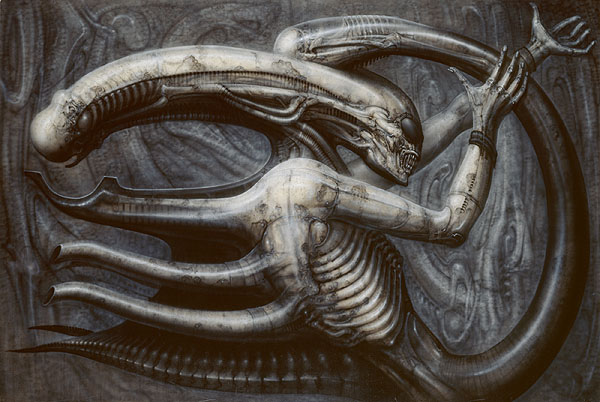The image depicts a highly detailed and intricate engraving that appears as a decorative feature on a metal door. Dominating the artwork is a long, cylindrical creature resembling an earthworm with distinct, alien characteristics. The creature's head is elongated, accounting for almost half the length of the image, and features large, black, lizard-like eyes and an open mouth with sharp, snarling teeth, giving it an aggressive expression. Emerging from the left side of its head are multiple tentacles. 

Moving along its body, which has a prominent rib cage structure that appears to be made of bone, the creature transitions into an unexpected human form. On the right-hand side, it has two human-like arms and hands, which are raised in an upward position. The hands are detailed and open, showing all ten fingers clearly. Adding to the surreal nature of the image, the creature's overall posture and placement in the artwork make it appear as if it's in a dynamic struggle with itself, reminiscent of an otherworldly being engaged in its own internal conflict. The artist's skill shines through the lifelike texture and depth, bringing this alien hybrid creature to vivid life.